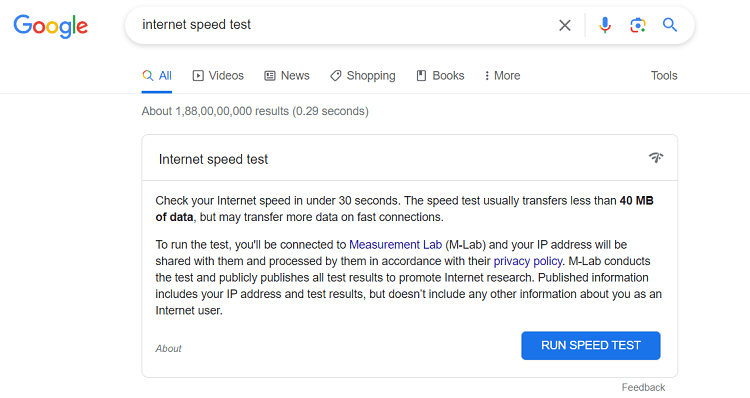The image features a colorful Google logo at the top left corner. Below it lies a prominently displayed rectangular dialog box with bulging sides, labeled "Internet Speed Test" on the left side, and an "X" icon on the right for closing the box. Within this box, there are icons, including a microphone, a potentially camera-like symbol, and a magnifying glass.

Under this dialog box, there's a navigation bar with various options. The word "All" is underlined in blue. To its right, there is an icon resembling a square with an arrow pointing right, labeled "Videos". Next, there’s a square icon with multiple lines, labeled "News", followed by a tag labeled "Shopping", and an icon of a page with a bookmark, labeled "Books". Three vertically aligned dots with the label "More" appear next, and finally, on the far right, the word “Tools” is displayed.

Below the navigation bar, the number of search results is indicated. A lightly outlined gray rectangle appears beneath this, containing text that starts again with the words "Internet Speed Test" beside a Wi-Fi symbol with a line through it. The text includes several black and bold (darker) fonts interspersed with blue hyperlinks, followed by a gray line with additional black text.

At the bottom of the gray rectangle, there is a prominent blue button labeled "Run Speed Test", and a smaller "Feedback" link directly under it.